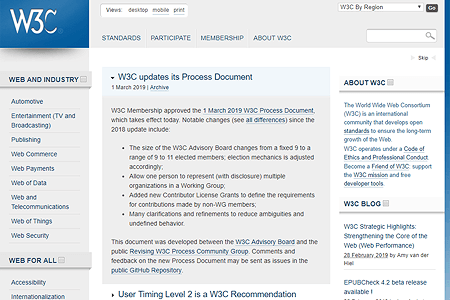The image is a slightly blurry rectangular screenshot with a gray background and blue and black text elements. In the upper left corner, within a blue box, the "W3C" logo is prominently displayed. Adjacent to this on the top navigation bar are the headings "Standards," "Participate," "Membership," and "About W3C," alongside a search bar located towards the right.

On the left side of the image, there's a vertical menu listing various categories: "Web and Industry," "Automotive," "Entertainment," "TV and Broadcasting," "Publishing," "Web Commerce," "Web Payments," "Web of Data," "Web and Telecommunications," "Web of Things," and "Web Security."

Centered in the image is an update titled "W3C Updates Its Process Document, March 1st, 2019." It announces that the W3C membership approved the March 1st, 2019 W3C Process Document, which is effective immediately. The update mentions notable changes, with a highlighted change being the size of the W3C Advisory Board, which now ranges from a fixed nine members to a variable nine to eleven members. The phrase "See all the differences" suggests that there is more detailed information available regarding these changes.